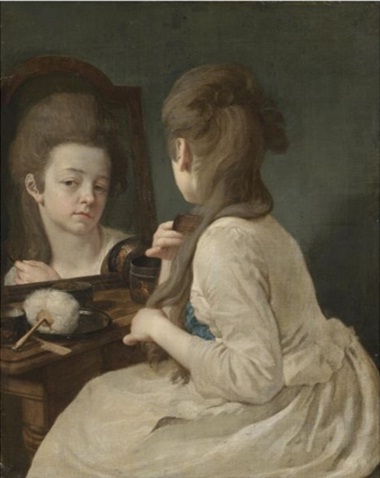This vertical rectangular image, sepia-toned with a dark background, portrays a woman sitting at a vanity, seen both from behind and in the reflection of a mirror in front of her. The image, which appears to be a detailed painting or photograph, exudes an old, nostalgic feel. The woman has long brown hair, part of which is piled up in a bouffant style while the rest cascades down to her waist. She's clothed in a white or light beige gown with a full skirt. Her face, framed by dark eyes, dark eyebrows, a small pointed nose, and thin lips, looks somewhat absent-minded or unhappy as she gazes into the mirror. Beside her on the vanity, which is made of dark wood and features a similarly framed mirror, are various items such as a cotton puff, pots, and a comb with a rat tail handle. The entire composition, highlighted by its antique sepia tone, gives a sense of quiet melancholy as the woman engages in the simple act of combing her hair, reflecting an intimate, solitary moment.